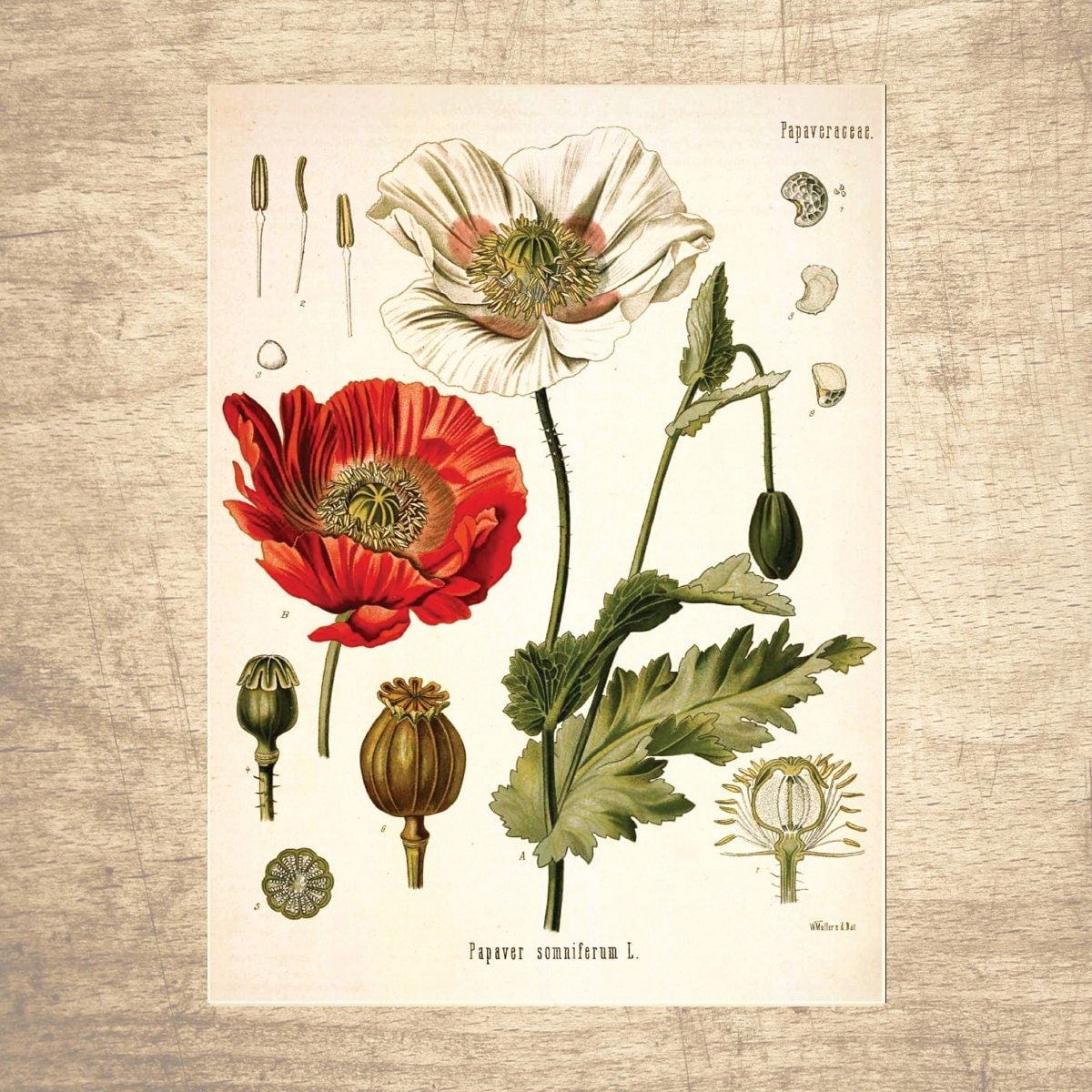This is a large square image, resting on a light brown wooden surface marked by both horizontal grains and vertical scratches. At the center of the image is a vertical rectangular sheet of paper or poster in a light beige or cream color, similar to parchment. The top of this paper features the text "Papa Veraci" in both the upper left and upper right corners. The focal point of the illustration is a detailed botanical diagram, prominently displaying a tall stem that extends upwards and curves slightly. At the top of this stem is a white flower with green seeds at its core and delicate pink spots around them. 

To the lower left of this main flower, another red flower with a brown center and a part of a green stem can be seen, adorned with large green leaves. Small water droplets are depicted above this red flower. Scattered throughout the illustration are additional green stems with flowers in various stages of blooming, represented by unopened bulbs in bronze hues. The bottom of the poster, centered beneath the illustration, is inscribed with the name "Papa Vera Somniferum L." This highly detailed botanical illustration combines elements of elegance and natural beauty, depicting various stages of flower development against a subtle and textured background.